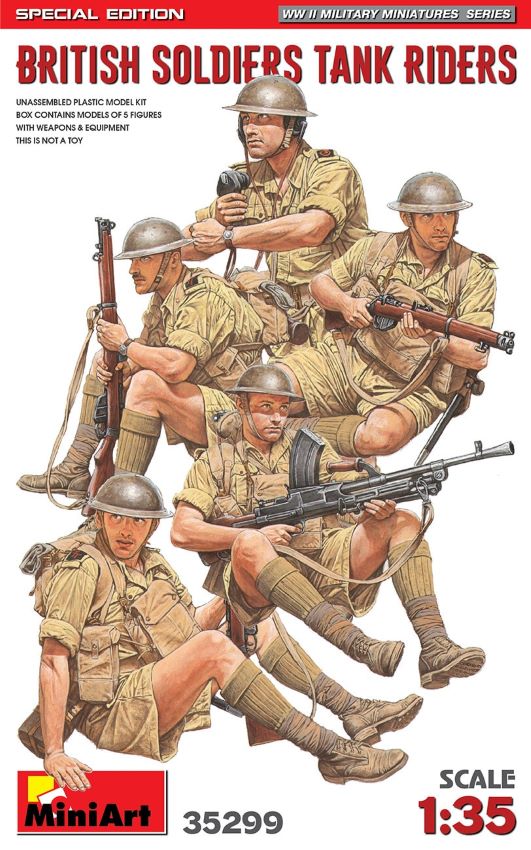This colored, artistic drawing depicts five British soldiers from World War I, identifiable by their distinctive helmets. They are seated in various positions, attired in khaki sand-colored uniforms suitable for a warm climate, characterized by boots, long socks, shorts, and short-sleeved shirts. Each soldier is equipped with wooden stock rifles, with one holding what appears to be a Thompson submachine gun. This unassembled plastic model kit, titled "Special Edition: World War II Military Miniature Series," features the British Soldiers Tank Riders at a 1:35 scale, and is marked with the identifier Mini Art 35299. The packaging includes details such as a red bar at the top with "Special Edition" in white lettering, and further descriptions in black and gray letters, indicating that this kit is for modeling purposes and explicitly stating it is not a toy.